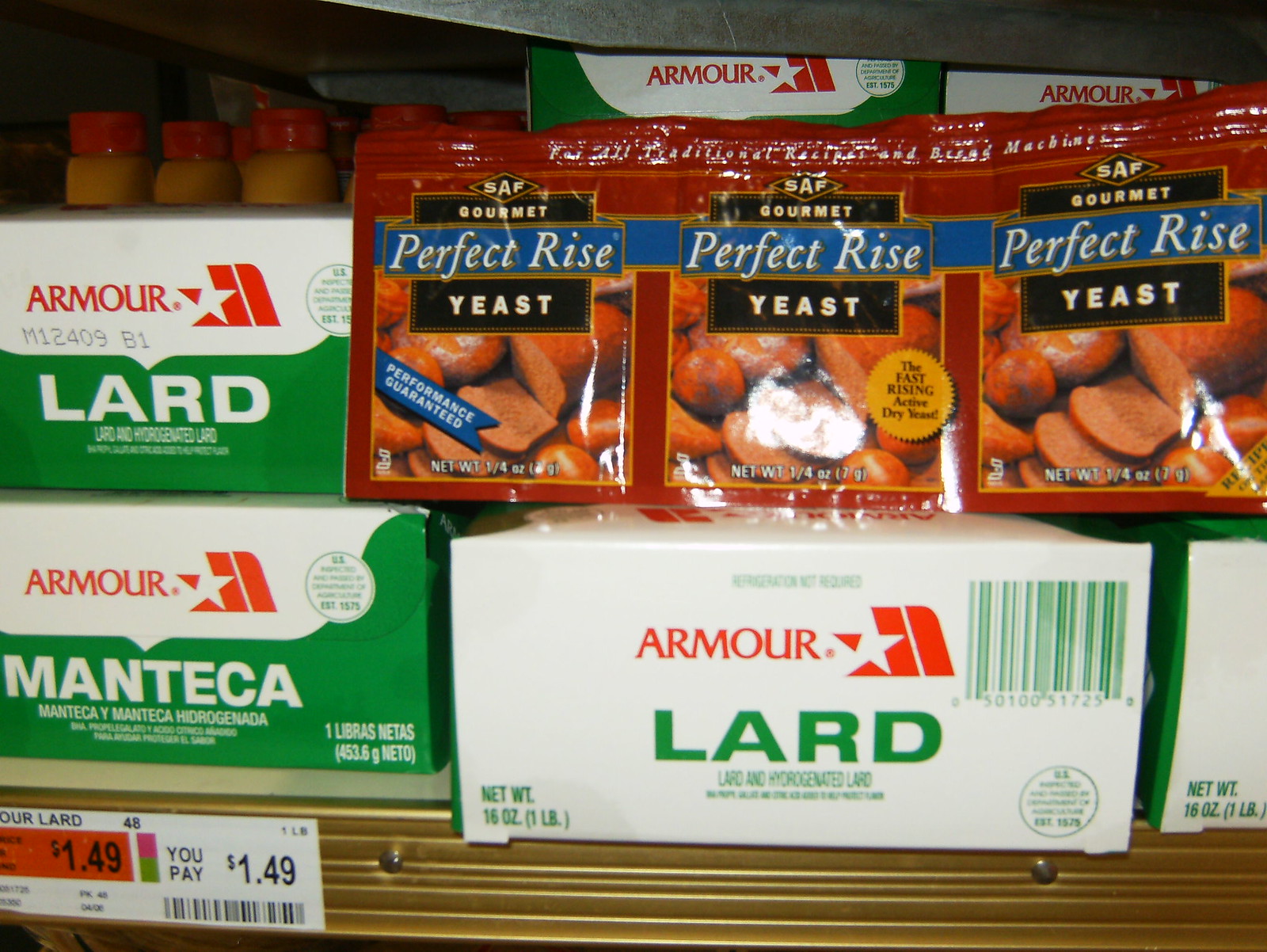The image showcases a collection of grocery items. Prominently displayed are three packets of SAF yeast products, each labeled differently: "SAF Gourmet Perfect Rice Yeast," "Performance Guaranteed," and "Fast Rising Active Dry Yeast." The packet descriptions mention a net weight of 1/4 ounce (7 grams). To the left and below these yeast packets are products labeled "Armour Lard," consisting of lard and hydrogenated lard. The pricing for the Armour Lard is clearly marked at $1.49, with a net weight of 16 ounces (1 pound). All items are neatly arranged on what appears to be a grocery holder or divider. Pricing information for the yeast products is not visible in the image.